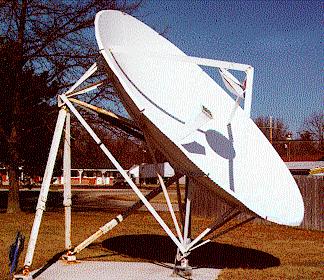The photograph captures a large white satellite dish mounted on a weathered white metal frame, set on a gray concrete pad amidst a lawn of dead, brown grass, indicating an older, somewhat vintage scene. The satellite dish is angled towards the upper right corner, with its clean white surface contrasting against the clear medium blue sky above. Shadows cast by the bright sunlight confirm the sunny weather. To the left, a green tree stands beside a weathered brown tree trunk, beyond which leafless trees suggest a fall or winter setting. In the background, multiple vehicles and another house add depth to the residential neighborhood scene. To the right, a heavily weathered wooden fence borders the area, enhancing the rustic feel of the image.